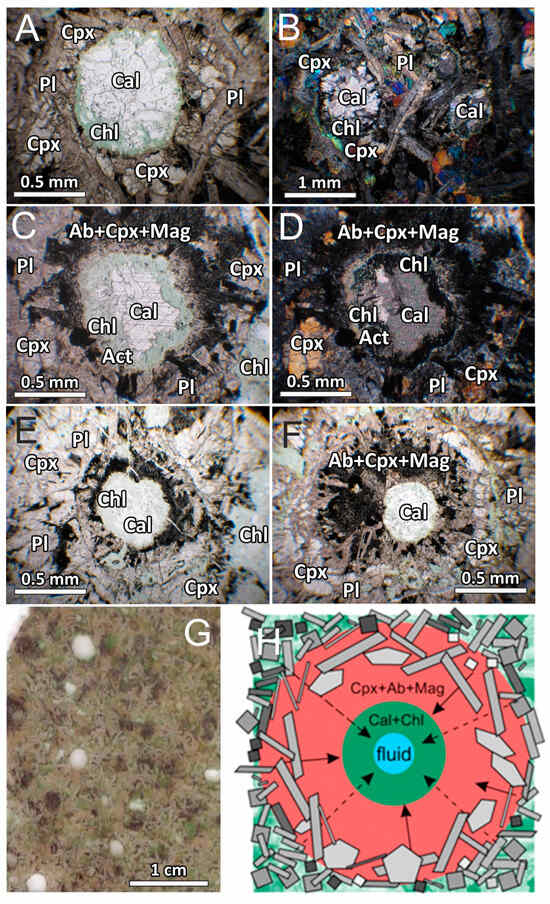The image is a scientific figure composed of eight micrographs arranged in four rows, each containing two images, labeled A through H. Each micrograph displays detailed observations under a microscope at various magnifications, indicated by the measurement scales of 0.5mm to 1mm. The images predominantly feature rock or crystal formations in different colors and textures, with recurring labels such as CPX (Clinopyroxene), PL (Plagioclase), CAL (Calcite), CHL (Chlorite), AB (Albite), and MAG (Magnetite). 

- **A**: Depicts a muddy area with concentric white circles and labels such as CPX, PL, CAL, and CHL scattered around.
- **B**: Shows a small landfill-like area with distinct colors, including blue and white, and similar labels.
- **C**: Displays a volcanic concrete-like texture with a prominent white central area and various mineral identifiers.
- **D**: Features a black charred surrounding with a central grayish-white region, again labeled with similar mineral abbreviations.
- **E**: Shows a predominantly white rocky area.
- **F**: A moon-like surface with a white center.
- **G**: Resembles a spongy or bubbly surface with dirty-looking bubbles.
- **H**: Contains a diagram with multicolored shapes transitioning from red to green to blue regions, labeled with CPX, AB, MAG, CAL, CHL, and "fluid."

The consistent labeling across images suggests a comparative study of the mineral content or composition across different samples or conditions, captured through microscopic analysis possibly related to geological or material science research.